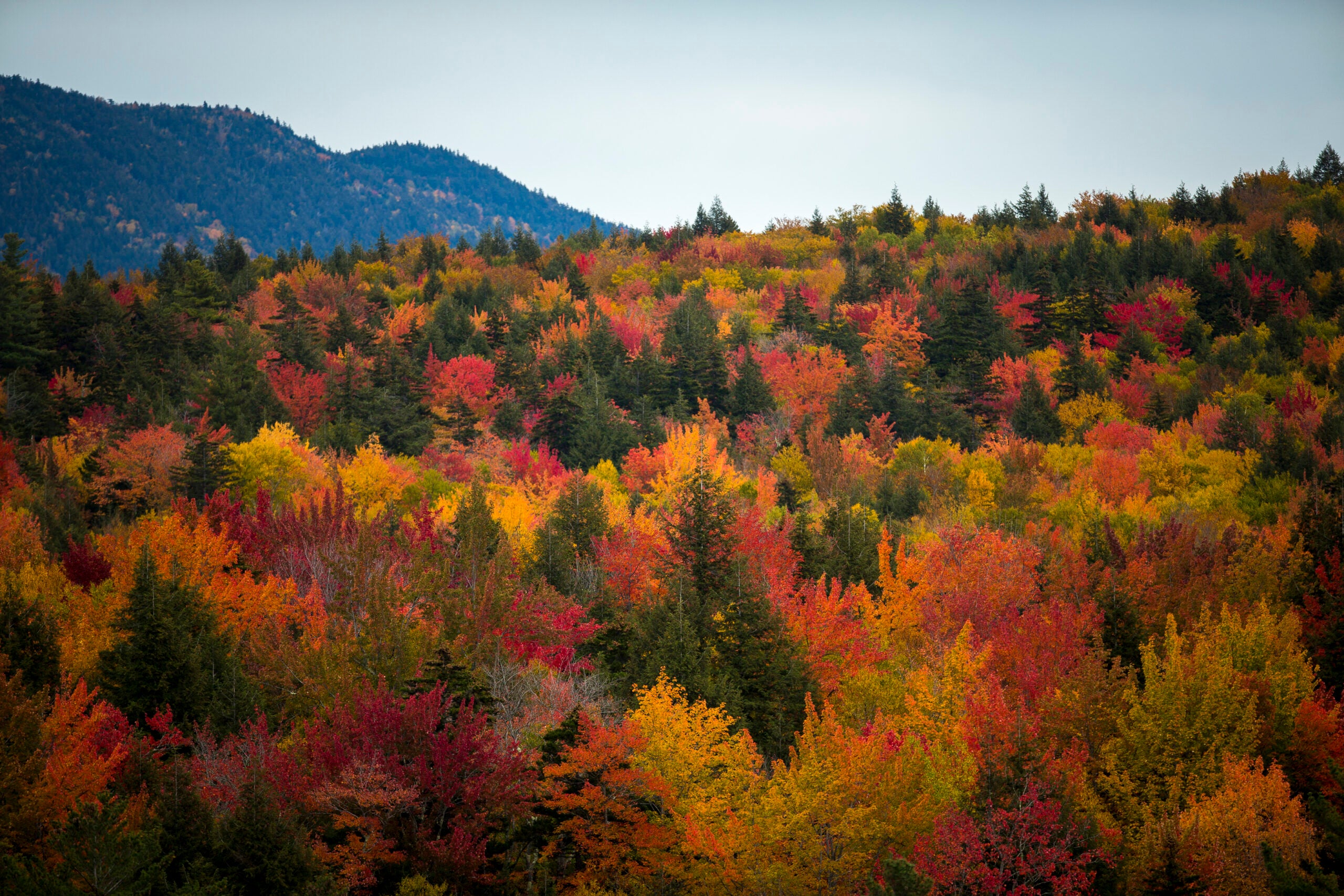This idyllic image showcases a vibrant autumn forest from an aerial perspective, captured during daytime under a predominantly blue sky accented with occasional white and gray hues. Dominating the scene are diverse trees, predominantly pine, interspersed with vibrant autumn foliage displaying a rich palette of yellow, red, and orange hues. In the foreground, the trees are closer, revealing a detailed spectrum of colors such as yellow, green, orange, red, and even pink. To the far left, distant hills are adorned with green trees, hinting at a possible valley between them and the colorful forest below. The middle and right portions offer a mix of sky and treetops, with the top left blending into the distant hills under the expansive, mixed-tone sky. This aerial view beautifully captures the essence of a tranquil fall day amidst nature.